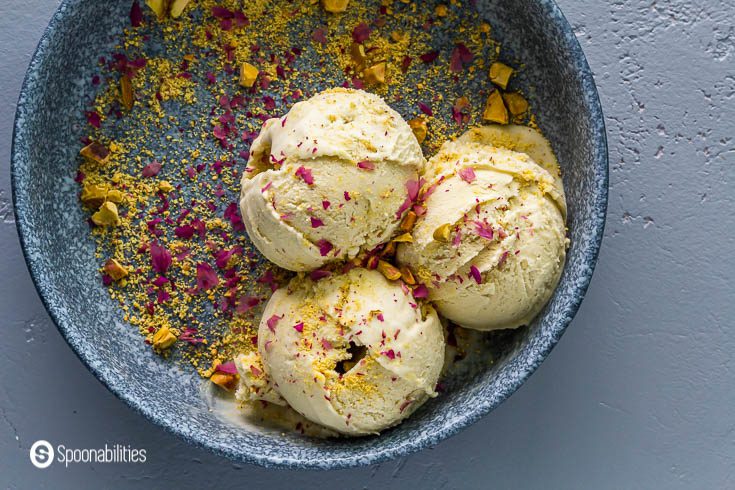The image features a bowl of three scoops of ice cream, set against a blue-gray background. The bowl, made of ceramic or stoneware, has a dark blue base with light blue spots, and it sits on a pale blue painted plaster surface, possibly resembling a concrete table. Each scoop of pale yellow ice cream is adorned with a mix of red and orange crumbles, resembling intricate seasonings or perhaps dehydrated flower petals. There are also small flecks of yellow powder and scattered chunks of pistachios, adding touches of green and orange to the overall presentation. The ice cream is sprinkled with these toppings not only on top but also around the bowl in an artistic manner, creating a visually appealing contrast with the bowl’s pattern. In the bottom left corner of the image, a white logo featuring an oval with the letter 'S' and the word “Spoonabilities” is displayed, seamlessly blending into the blue-gray background.